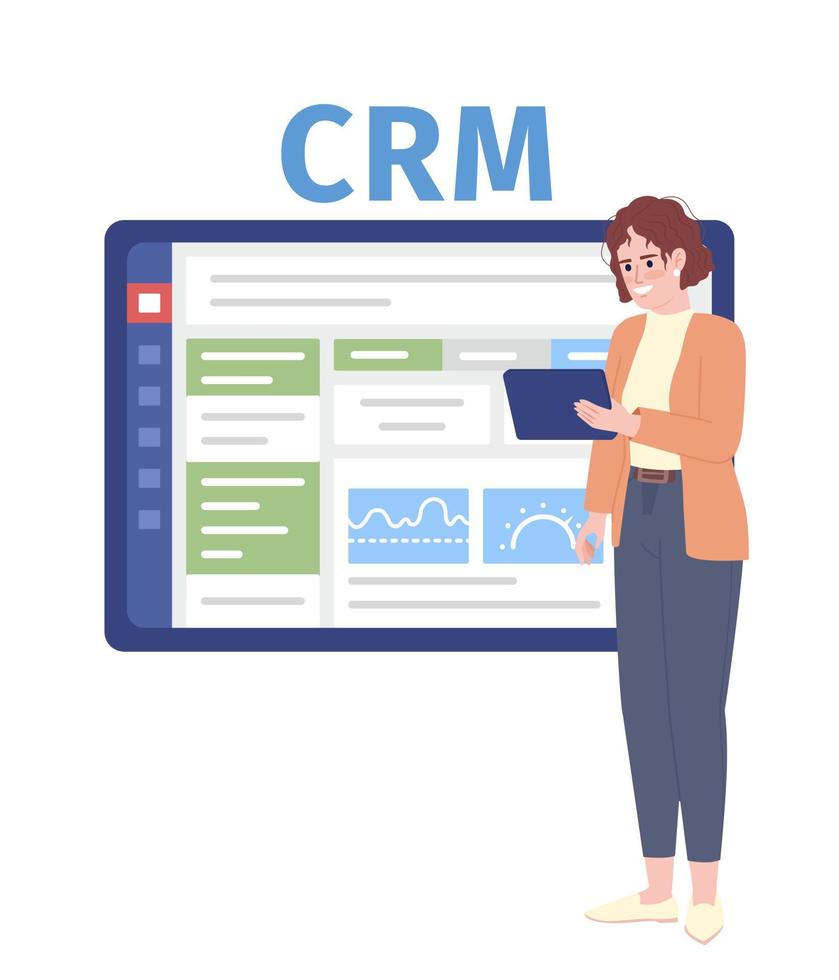The image depicts a cartoon-like drawing of a woman standing against a solid white background. She has chin-length wavy brown hair and is wearing blue pants with a brown belt, a yellow shirt, an orange long-sleeved cardigan, and cream-colored shoes. Her right arm hangs down to her side, while her left arm is bent at the elbow, holding a blue electronic pad, which could be a book or an iPad. To her left, there is a large tablet-like screen, approximately three to four inches wide and two to three inches high, with the letters "CRM" displayed at the top in large blue print. The screen is bordered with beveled edges and contains various icons and buttons in colors such as red, green, light blue, white, and gray. The background remains plain and white, with no visible borders, emphasizing the central focus on the woman and the screen.